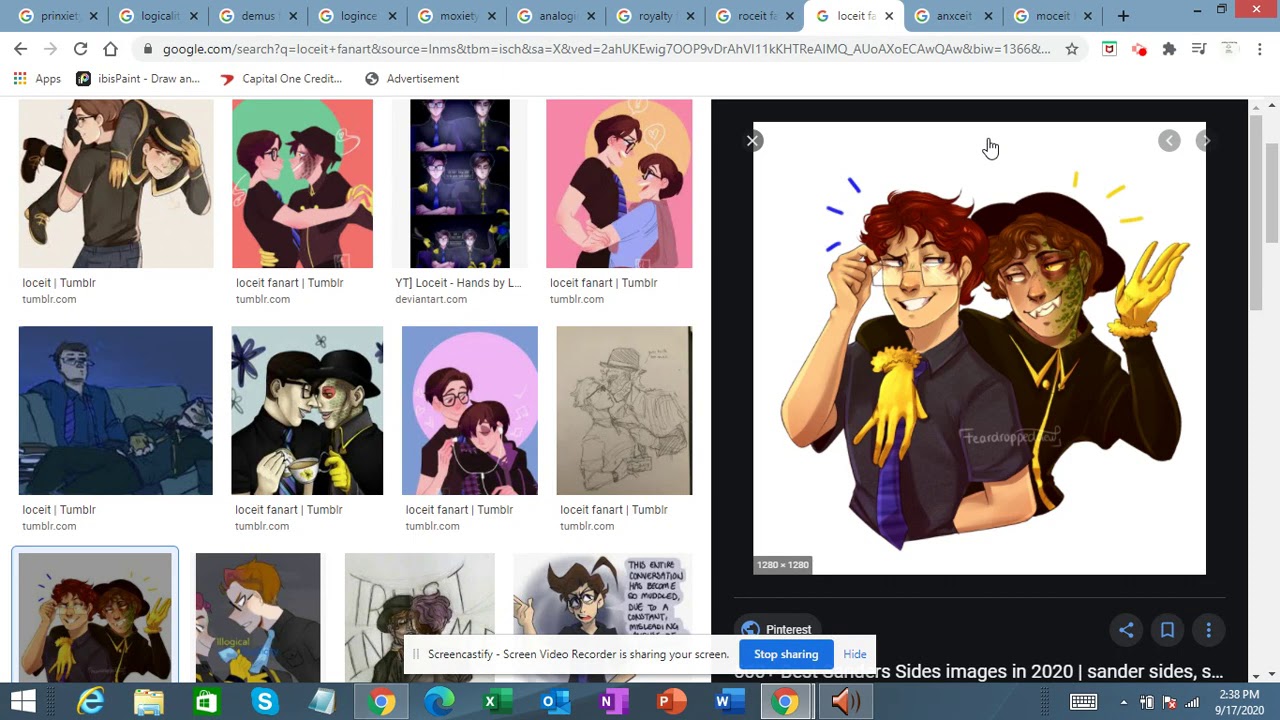The screenshot is highly detailed and cluttered. Spanning horizontally across the screen is a blue-gray rectangle, indicating a busy workspace with numerous unreadable tabs open at the top. In the upper right-hand corner, a small rectangle featuring a white 'X' is visible, presumably for closing a window or application. Below this area, the browser's address bar is situated, complete with navigation buttons—right and left arrows, a home icon, and a reload button.

On the left side of the screen, there are three rows each containing four computer-generated images. To the right of these images is a large black square, undefined in its purpose. Above this, a white square presents a computer-generated image of a man, resembling a scarecrow with an arm around him.

At the very bottom of the screen is another blue-gray rectangle, similar in color to the one at the top. This lower rectangle serves as a taskbar, displaying various icons and applications such as Chrome and Explorer. The screen also features dual scroll bars on the right, indicating a substantial amount of content available to navigate.